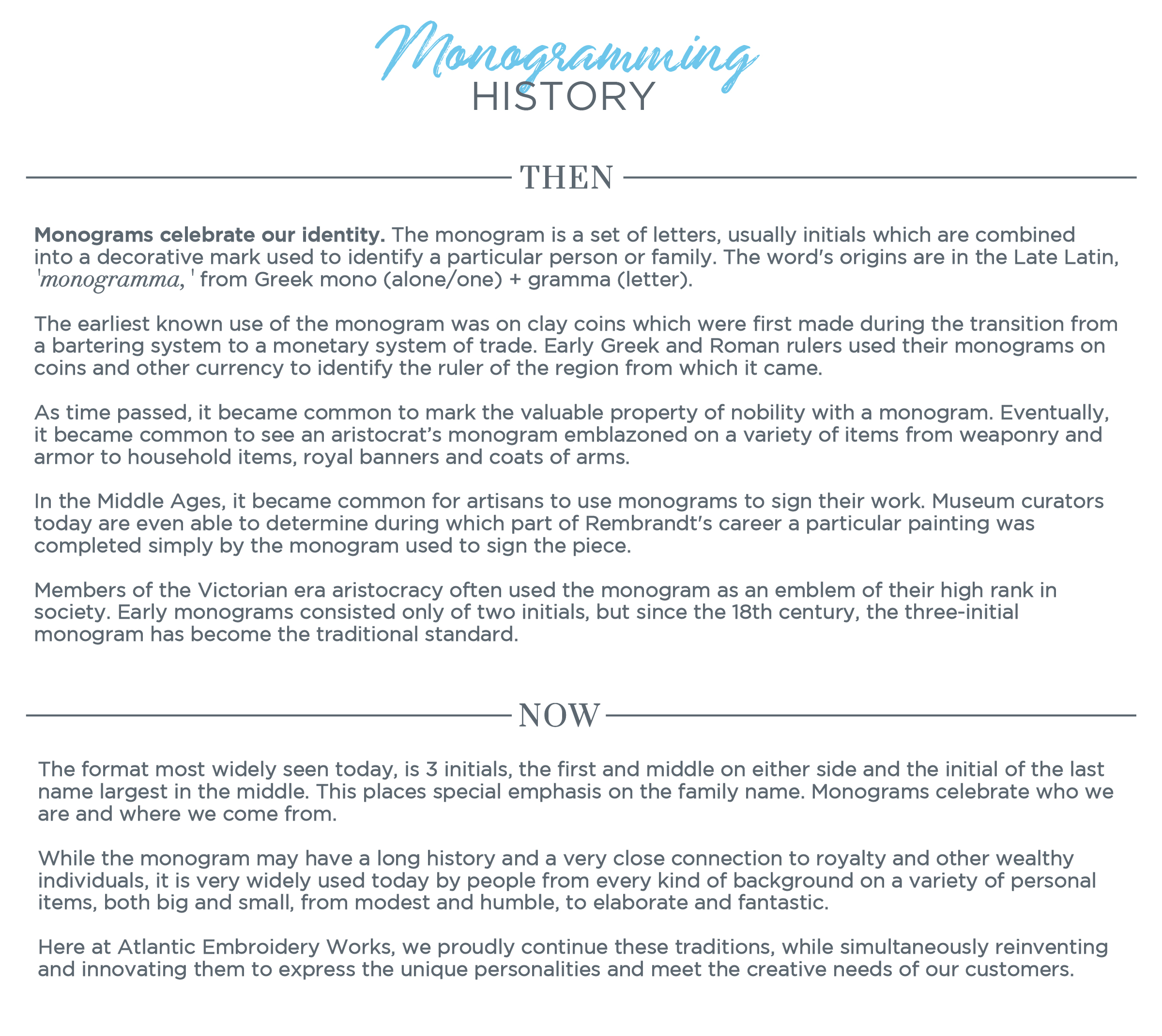The image appears to be a webpage dedicated to the history and modern adaptations of monogramming. At the top, the title "Monogramming History" is elegantly written in blue cursive. The main body is composed of dense black text that delves into the evolution and cultural significance of monograms. It explains that a monogram is a set of letters, typically initials, combined into a decorative mark to identify a particular person or family. The term originates from the late Latin "monogramma," derived from Greek "mono" meaning "alone" or "one" and "gramma" meaning "letter."

The earliest monograms were found on clay coins, emerging with the shift from bartering to monetary systems in ancient Greek and Roman societies. These early monograms signified the ruler of the currency's region. Over time, monograms became an emblem of nobility, marking valuable possessions, weaponry, armor, household items, royal banners, and coats of arms. By the Middle Ages, artisans began using monograms to sign their works.

Today, the widely recognized format features three initials: the first and middle initials on either side, with the last name's initial larger and in the center, emphasizing the family name. Monograms continue to celebrate identity and heritage and are now accessible to diverse audiences, appearing on various personal items like hats, coats, mugs, and more.

Atlantic Embroidery Works remains committed to these traditional practices while innovating to reflect the unique personalities and creative needs of their customers. Monograms thus not only showcase our origins but also express individuality across time.